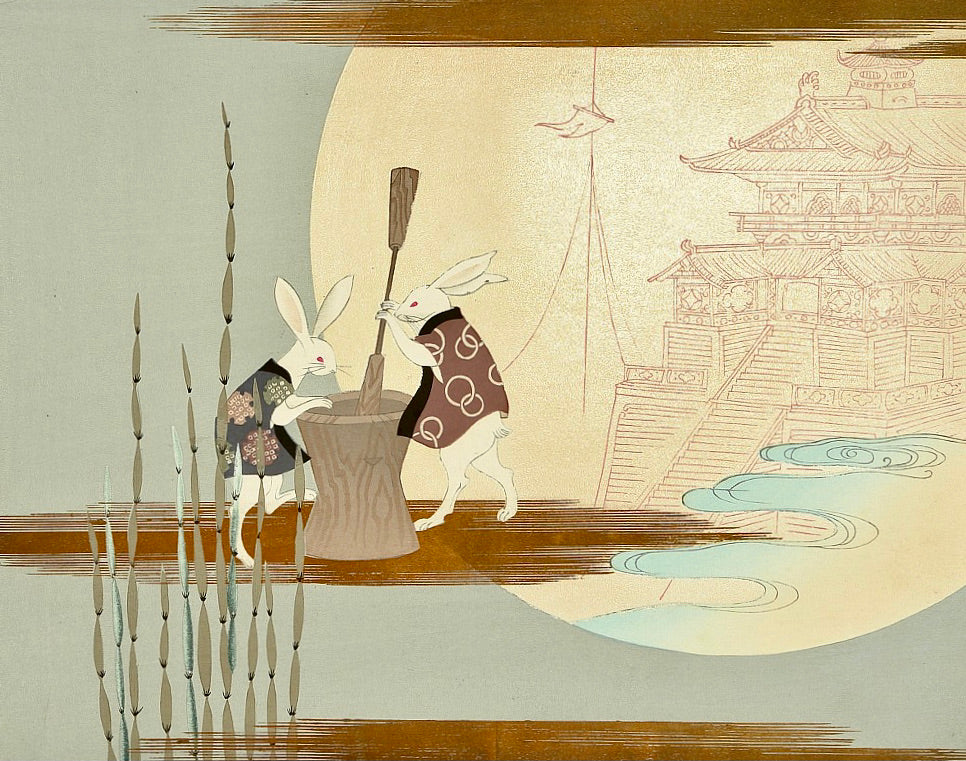This intricate art drawing features two anthropomorphic white rabbits with red eyes, both dressed in traditional short kimonos. They stand on their hind legs beside a large wooden cauldron, appearing to mix its contents with a wooden paddle. The rabbit on the left wears a gray kimono adorned with floral patterns and black trim, resting its paws on the cauldron’s edge. Its companion, slightly taller and on the right, dons a reddish-gray kimono with interlocking circle motifs and also black trim, actively stirring with the paddle. The cauldron itself is gray with light reddish lines resembling wood grain and narrows at the middle, giving it a distinctive shape.

The rabbits are set against a background featuring a classic Asian theme. To their right looms a grand pagoda or possibly an imperial palace with multiple levels and steep, A-framed roofs. The structure, intricately etched into the scene, is flanked by blue swirls hinting at water, adding a dynamic element to the composition. The background is dominated by a large, glowing, yellowish-white moon that envelopes the scene, casting a serene light over the entire drawing. In the foreground, bamboo shoots grow from the left side, partially overlapping the left rabbit, and horsetail reeds add an additional layer of depth to the artwork. The landscape and calm, pastel colors, primarily light gray and blue, enhance the peaceful and meticulous Asian-inspired sketching style.